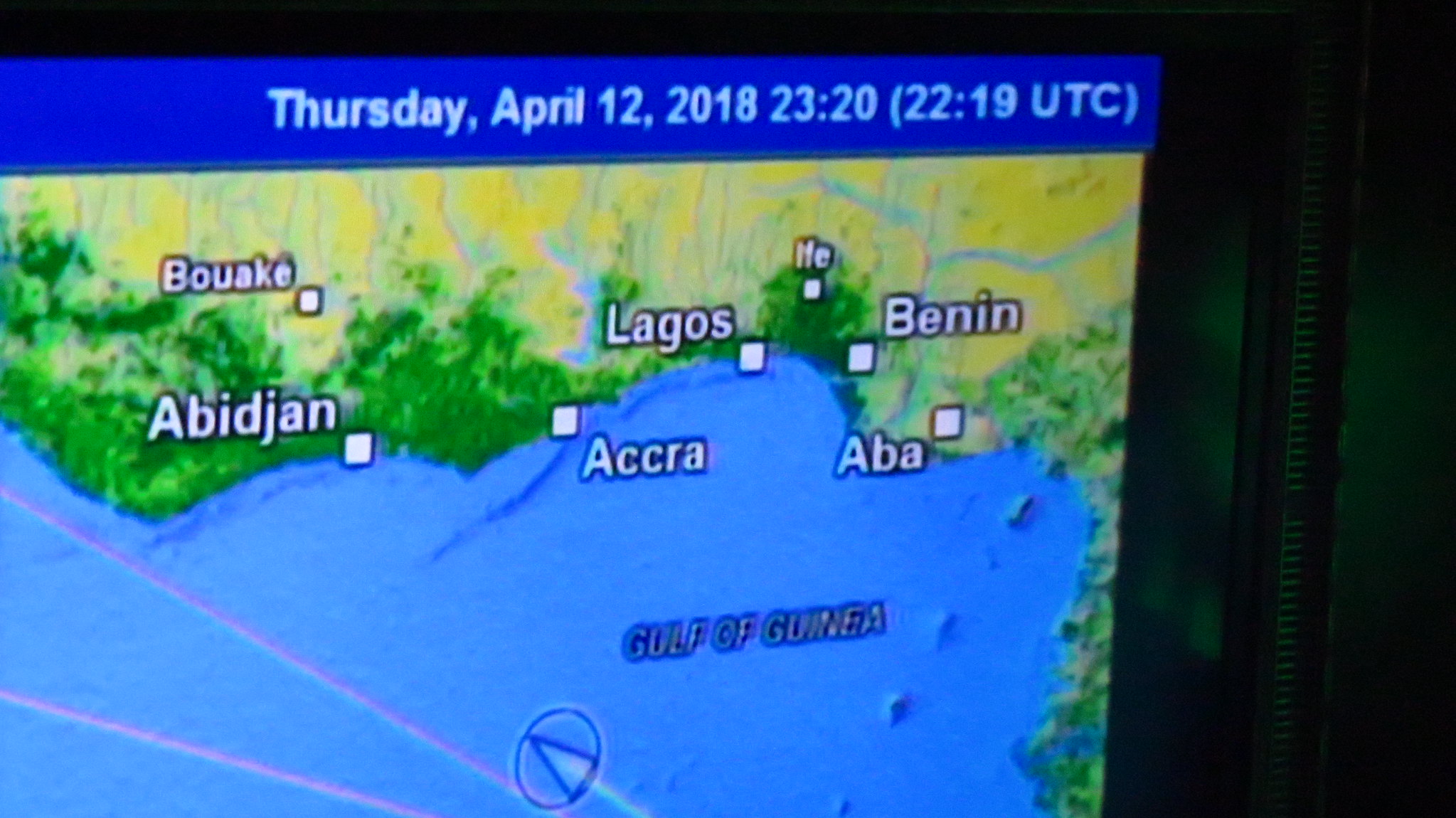The image depicts an indoor scene with a prominent screen, possibly from an airplane, a television, or a computer monitor, set against a black background. At the top of the screen, there is a dark blue strip with white lettering displaying "Thursday, April 12, 2018," along with the time "23:20 (2219 UTC)." Below this, the screen showcases a detailed map. The map features land areas in yellow and green, indicating possibly different terrains such as forests and plains. The blue areas represent bodies of water, with the Gulf of Guinea labeled at the bottom right. Visible locations on the map include Buake, Abidjan, Lagos, Accra, Ife, Benin, and Abba. Additionally, there are directional arrows pointing towards the left side of the screen.